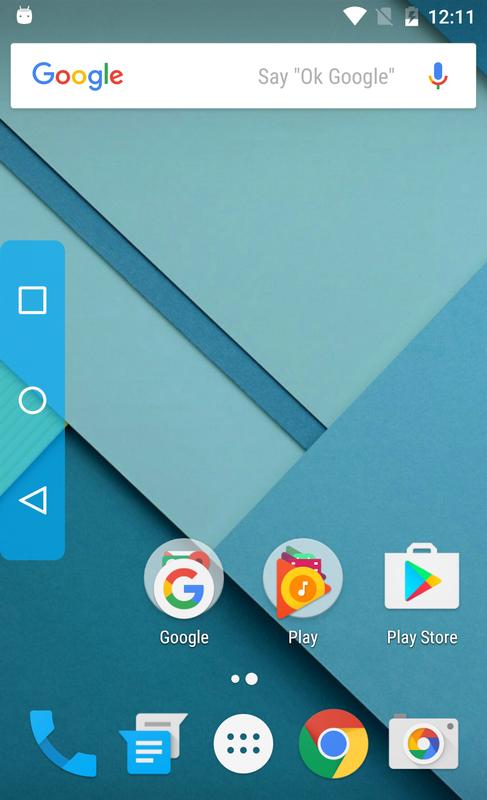Descriptive Caption:

The image depicts a smartphone home screen with a colorful geometric wallpaper. The background features a gradient of blue shades, starting with a darker blue in the bottom left, transitioning to a medium blue to the right, and culminating in a very light blue with a diagonal strip running through it. At the top of the screen, the time is displayed as 12:11, and the battery icon shows it is charging with a lightning bolt symbol.

Prominently placed at the top center is the Google search bar, identifiable by the rainbow-colored Google logo and a blue microphone icon to its right. Below the search bar and slightly to the left, there's a semi-transparent royal blue bar.

Towards the bottom of the screen, the typical app icons are arranged. On the left is the Google Play Store icon, followed by the phone call button, a messaging app icon, and the Google Chrome browser icon. Lastly, the camera icon is positioned to the left center of the screen. In addition, there's a white circle with a series of dots within it, likely indicating the app drawer. The overall layout seems to be somewhat inverted, with elements like the square app icons being placed differently from the usual bottom alignment.